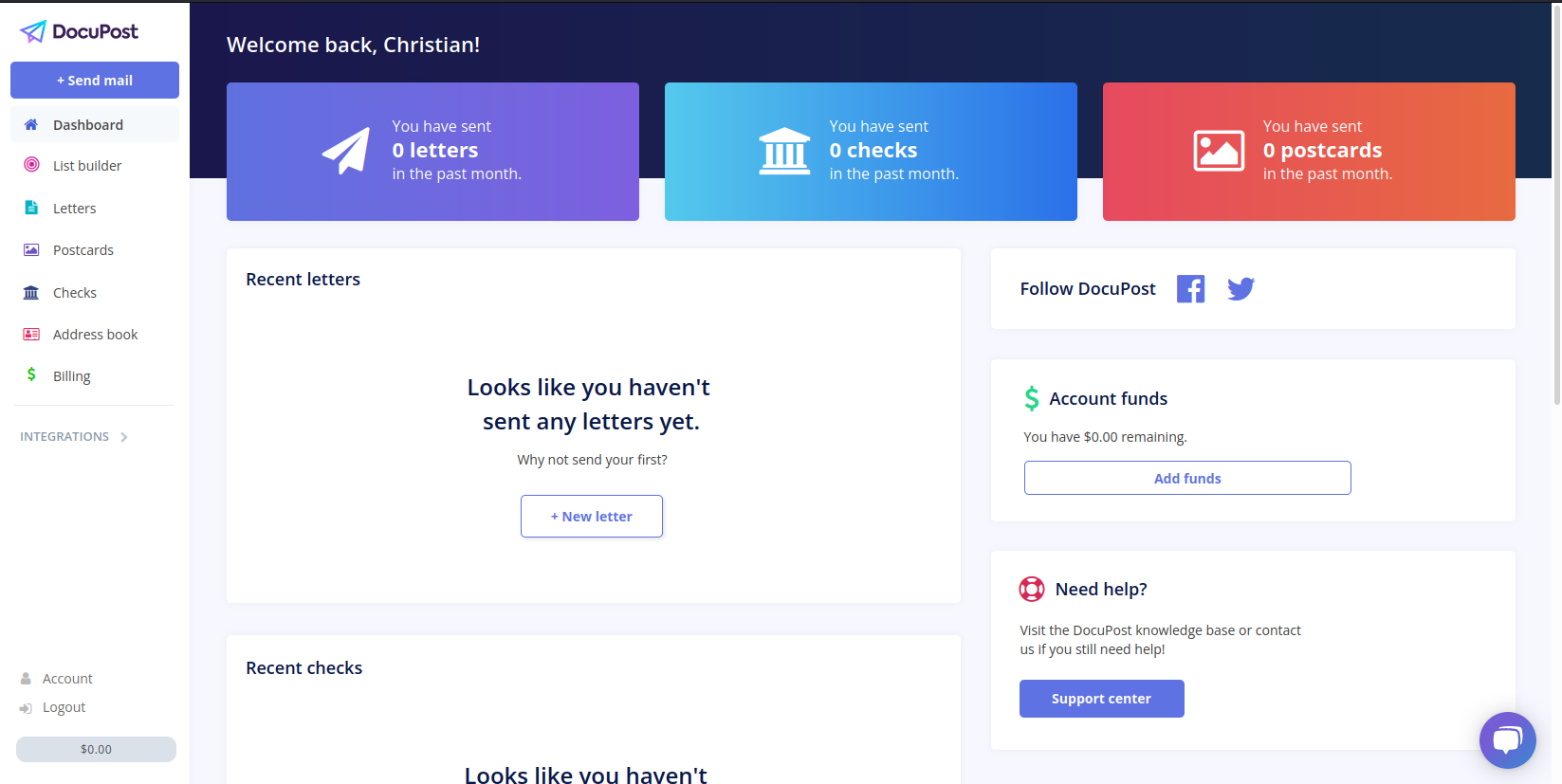A screenshot from the DocuPost web application showcases its user interface. On the left sidebar, the DocuPost title and logo—a paper plane icon pointing to the right—are prominently displayed at the top. Beneath it, there is a blue "Send Mail" button, followed by a navigational list featuring options such as Dashboard, List Builder, Letters, Postcards, Checks, Address Book, Billing, and an Integration section. At the bottom of the sidebar, users can access their account details and log out, with a grey button indicating a balance of $0.00.

In the main content area, a welcome message reads "Welcome Back," set against a black header. Directly below, three informational boxes are aligned horizontally: the first box is purple, stating that zero letters have been sent; the second box is blue, showing zero checks sent; and the third box is red, indicating zero postcards sent.

Further down, the interface features two main charts: "Recent Letters" on the left, and "Follow DocuPost" on the right, with accompanying Facebook and Twitter icons. Beneath these, a second row includes a chart titled "Recent Checks," followed by an account management section featuring an "Accounts Fund" display, an "Add Funds" button, and a "Need Help and Support Centre" button. The interface is clean and user-friendly, designed to facilitate easy navigation and efficient use of DocuPost's mailing and financial services.